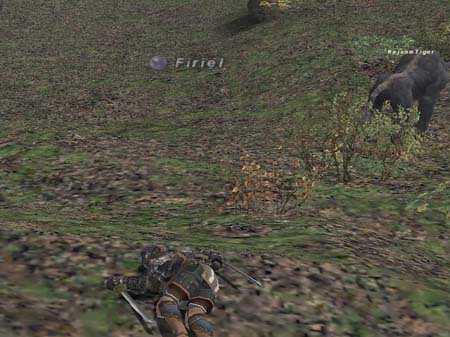The image depicts a rugged hillside strewn with a mixture of rocks and grass. A prominent boulder appears approximately halfway up the slope. Across the middle of the image, a small sign reads "Furial." Near the top of the hill, a black animal resembling a tiger with a distinct gray streak running from its shoulder down its back can be seen. At the base of the hill, the somber scene includes the figure of a deceased soldier, clad in armor and lying face down among the rocks, with a large sword lying beside him.